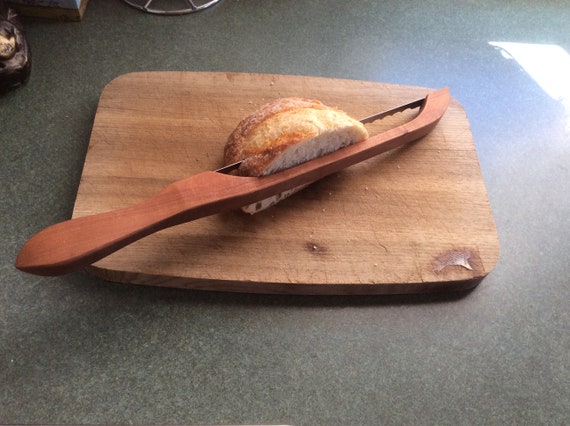The photograph depicts a scene on a dark gray Formica countertop with a distinct wooden cutting board placed at its center. The cutting board features horizontal wood grain and some visible grease stains and cut marks. A unique, wooden-handled bread saw with a straight blade is positioned on the board, actively slicing a small piece of golden-brown bakery bread. This bread knife has a distinctive design, where the handle is connected to the blade by a wooden frame, creating a gap through which the bread fits as it is being sliced. Light, likely from a nearby window, illuminates the scene from the top right corner. In the top left corner, there are several indistinguishable objects. The overall impression is of a quaint, sunlit kitchen moment, captured in detail.